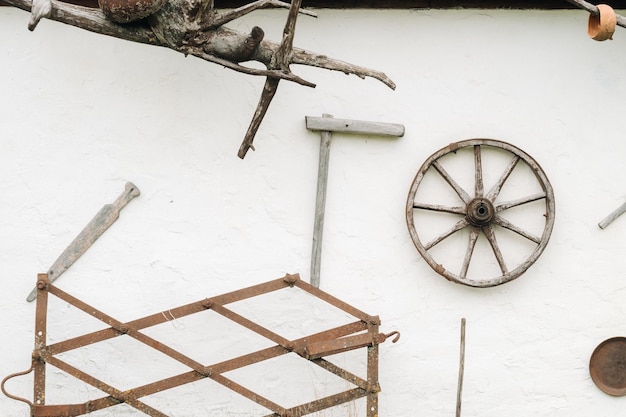The image showcases an eclectic outdoor display against a white stucco wall adorned with various vintage items. Dominating the wall is a gnarly, branched piece of driftwood in the upper left corner, casting intriguing shadows with its knots and texture. To the right, near the upper corner, another tree branch is adorned with a ceramic bracelet, reminiscent of terracotta in color. Centrally positioned on the right half of the wall is a rustic wooden wagon wheel with nine spokes radiating from its center. Scattered around these larger items are smaller, weathered wooden paddles and knickknacks, including a wooden mallet. In the lower left corner, a rusted, brown metal trellis or collapsible gate crisscrosses down, partly obscuring what appears to be an old, handle-less saw blade. Lastly, nestled in the bottom right corner is a round, brass-like pan, heavily rusted, enhancing the antiquated charm of the scene. This collection of random but evocative objects sits propped against the textured, stuccoed wall, creating a picturesque vignette of nostalgic artifacts.